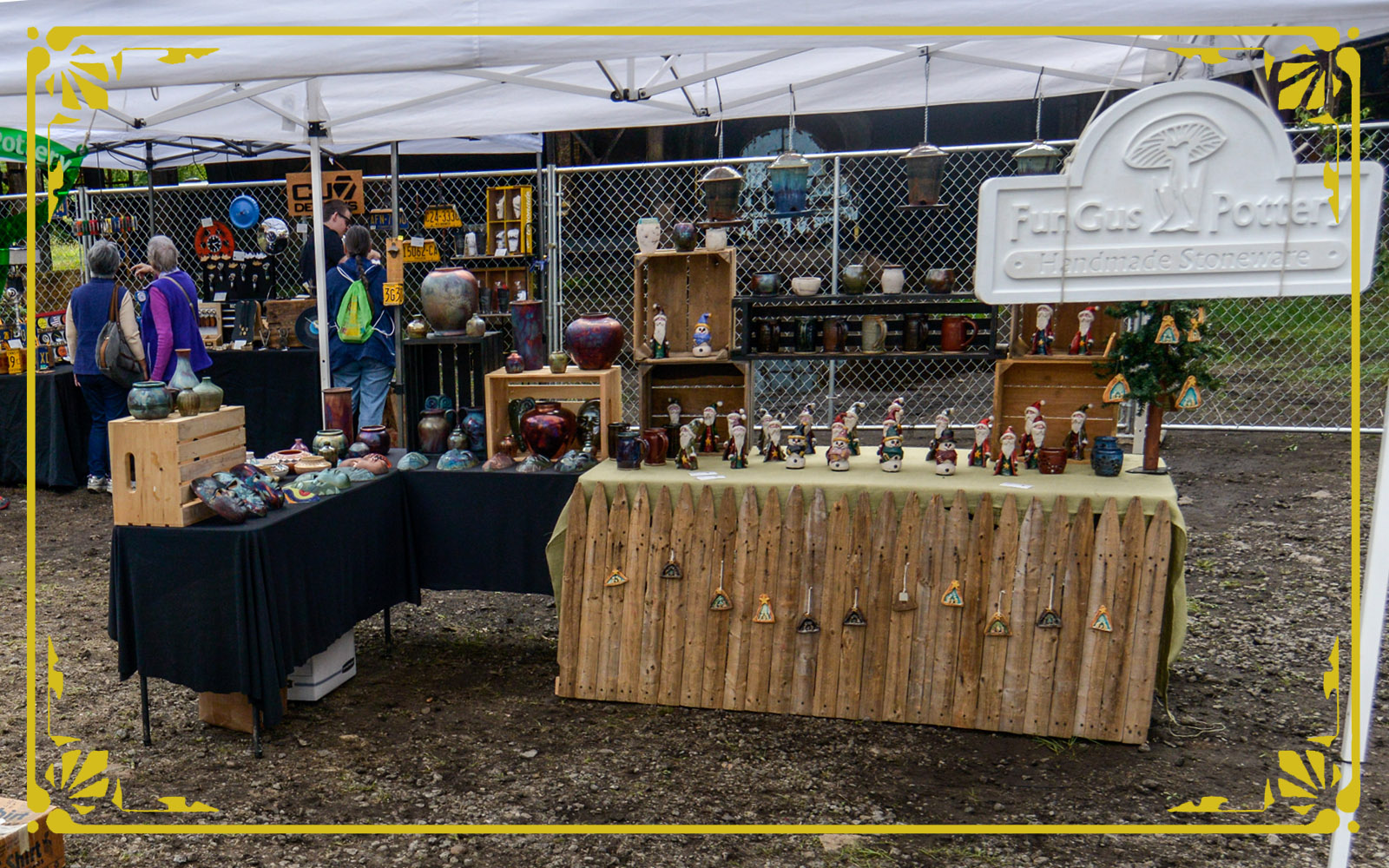The photograph depicts an outdoor vendor booth set up during the daytime, characterized by a white tent canopy. The image is bordered by a dull yellow frame with simple corner designs. The booth, positioned behind a six to seven-foot chain-link fence, is focused on an L-shaped table covered with a black tablecloth. Displayed on the table are a variety of small ceramic trinkets, including figurines resembling gnomes, Santa Claus, and snowmen, along with other pottery items like vases and cups. These items are elevated using wooden crates. In addition, there appears to be a section with hanging tree decorations in front of the table. Notably, in the top right corner of the image, there is a sign that reads "Fungus Pottery, Handmade Stoneware," featuring a small mushroom illustration. The area behind the table has gravel ground, indicating an outdoor setting, and on the left side of the image, people can be seen shopping at another booth.